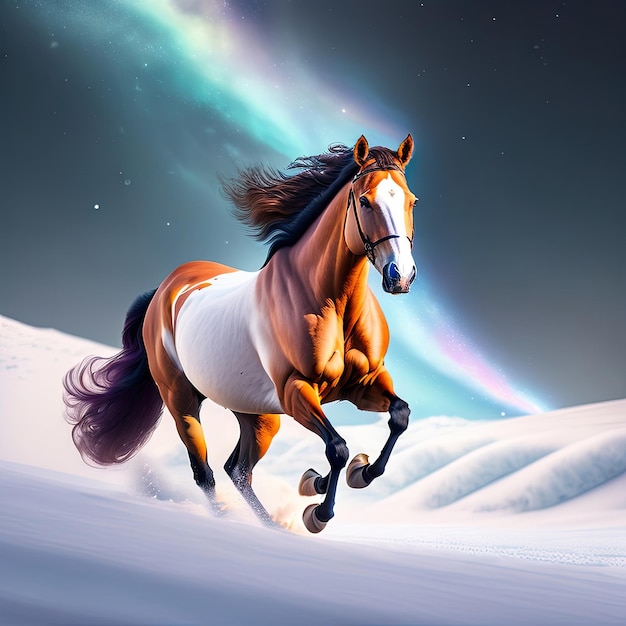The image depicts a captivating nighttime scene where a powerful and majestic horse is running through a snowy landscape. The horse is predominantly brown with a striking white blaze on its face, and its midsection and belly are beautifully white. Contrasting against the white of the snow and the horse’s markings, it has a flowing black mane and tail. The horse's muscular body exhibits an energetic pose with its front legs raised, exuding a sense of wildness and freedom.

In the background, the night sky is lit by an ethereal display of the aurora borealis, with colors transitioning from light blue to a deep black-blue, particularly intensifying at the top right corner of the image. The celestial scene is further enhanced by numerous stars scattered across the sky, contributing to the magical and serene atmosphere. 

The illuminated snow under the presumably full moon adds to the surreal quality of the image, making the horse appear almost mystical as it races through the snowy hills. The entire scene combines elements akin to a painting, emphasizing the horse's spirited nature and the dreamlike environment it inhabits.